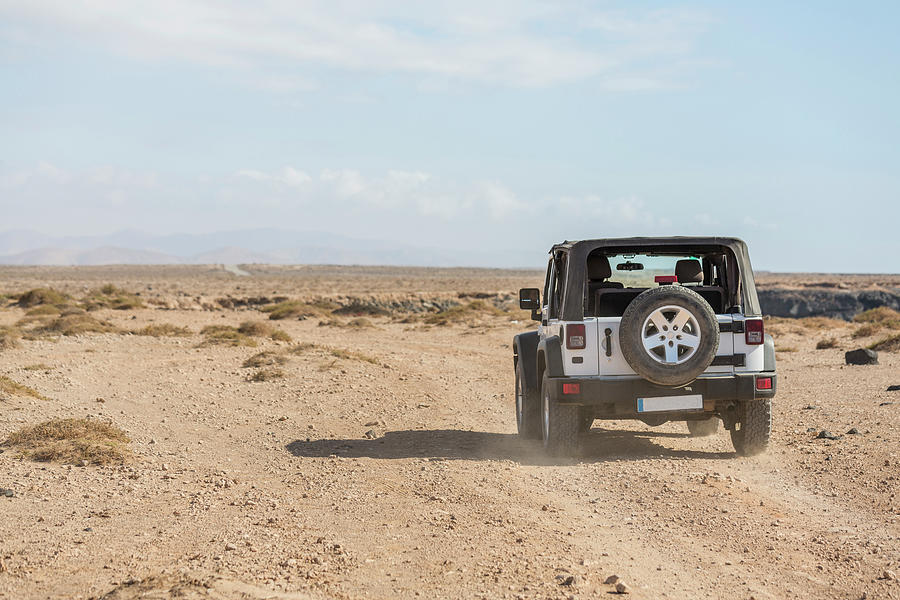In this image, a white, four-wheeled Jeep with a black soft top is navigating a dusty, desolate desert plane. Positioned in the foreground on the right side of the image, the vehicle features an exposed interior with gray headrests, no windows, and a spare tire mounted on the back. Tracking on a gravelly path lined with faint tire marks from previous vehicles, the Jeep is making its way into a stark, expansive landscape. The ground is predominantly beige and sandy, dotted with tufts of dead vegetation and occasional patches of sagebrush or twigs. The backdrop reveals a scarcely visible mountain range through a haze, extending towards a horizon that melds with a vast, blue-gray sky filled with thin, scattered clouds.